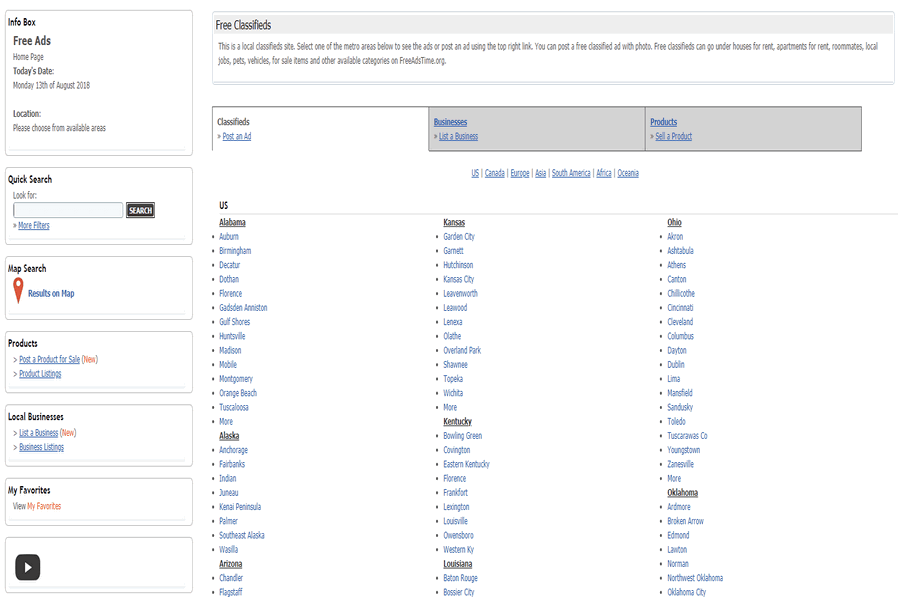The image displays a webpage with several distinct sections, organized to provide a comprehensive user experience for posting and searching classified ads. The background of the webpage is predominantly white, enhancing the readability of the black text.

**Top Left Section:**
- **Info Box:** This area features the heading in black text. Subsections inside this box include:
  - "Free Ads"
  - "Homepage"
  - "Today's Date: Monday, 13th of August 2018"
  - "Location: Please choose from available areas"

**Second Section (Directly Below the First):**
- **Quick Search:** This section is dedicated to a quick search feature. It includes:
  - A text field labeled "Looking for"
  - A black search button
  - A link labeled "More filters" in blue text

**Subsequent Sections:**
- **Map Search:** Contains options for searching results on a map, with the relevant text in blue.
- **Product:** Options for users to "Post a product for sale" and "Product listing."
- **Local Businesses:** Prompts for listing a business and exploring business listings.
- **My Favorite:** A section where users can view their favorites, with "My Favorite" highlighted in orange.

**Top Part of the Page:**
- **Free Classified:** A broad description indicating that this is a local classified site. Users are instructed to:
  - Select a metro area to see existing ads
  - Post an ad using the link provided at the top right
  - Post free classified ads with photos
  
  The free classified section also includes potential categories such as:
  - Houses for Rent
  - Apartments for Rent
  - Roommates
  - Local Jobs
  - Pets
  - Vehicles for Sale
  - Items
  - Other available categories found on FreeAdsTime.org

**Bottom Part of the Page:**
- **Classified Categories and Geographic Areas:** Users can post ads or list businesses and products across various regions. Categories and sections mentioned include:
  - US States (e.g., Alabama, Alaska, Arizona)
  - Continents and regions (e.g., Canada, Europe, Asia, South America, Africa, Oceania)

Beneath each US state, cities are mentioned and are listed in blue text, allowing users to easily navigate to specific local areas.

This well-structured layout ensures users can effortlessly find or post ads, search for products or businesses, and target specific geographic locations with ease.